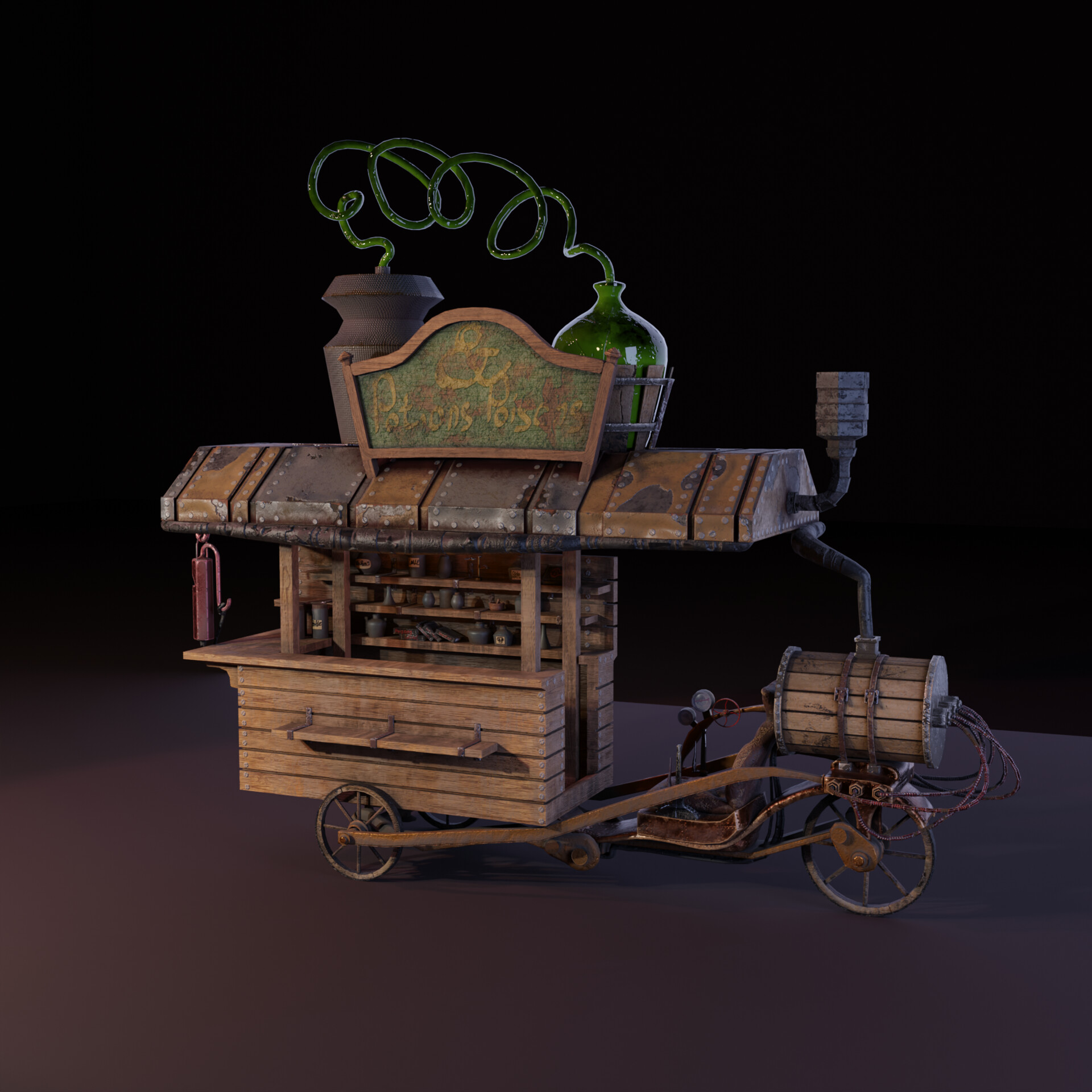A square, dark image depicts a wooden model of a vintage three-wheeled cart or food truck positioned centrally, facing right. The upper half of the background is solid black, with the lower half resembling a brown counter or table. The cart features a combination of brown and gray metal parts, including a corrugated roof that extends beyond the wooden shelves below. These shelves, designed for serving, display various brown and gray containers, resembling a portable bar or mobile store.

The front of the cart is mounted on a single wheel, with another wheel visible on the side and a presumed third wheel on the opposite side. At the front, a barrel with copper-colored bolts and poles sits atop the wheel. A small detailed figurine appears to operate the cart, adding character to the scene.

The top of the cart features a metallic roof, again in brown and tin or copper hues, with green and yellow signage. This roof covers a shelf area stocked with glassware and bowls. A green bottle with tubing connects to a cylindrical ornament, enhancing the model’s intricate display. The overall scene speaks to an era of hand-crafted mobile shops or bars, blending rustic aesthetics with a touch of whimsy and nostalgia.